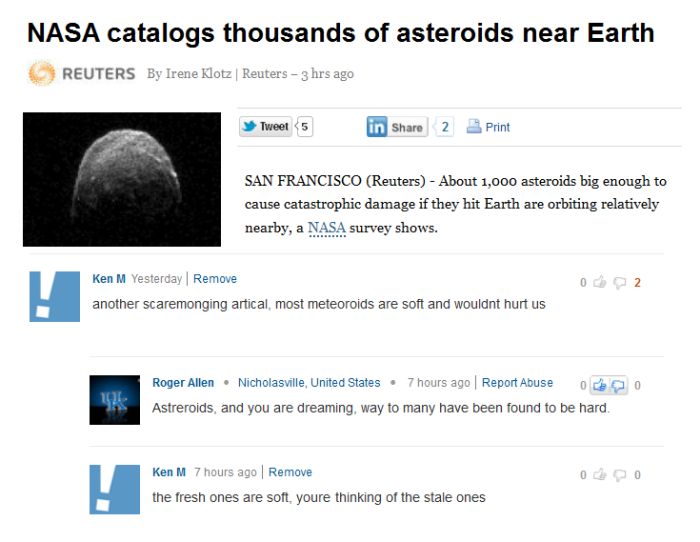**Descriptive Caption:**

A screenshot from a news website features an article titled "NASA Catalogs Thousands of Asteroids Near Earth" at the top in black text. Above this headline, an orange swirl graphic appears with the text "Ruckers by Aaron Klotz | Ruckerts - three hours ago." Centrally displayed is an image of a gray asteroid, set against a gradient background that transitions from bright at the top to dark at the bottom. Below the image are interactive options labeled “tweet, five,” “cheer, two,” and “print.”

The main body of the article begins with the dateline "San Francisco (Ruckers)" and reports that "about a thousand asteroids, big enough to cause catastrophic damage if they hit Earth, are orbiting relatively nearby, a NASA survey shows." 

Following the article, a comments section is visible. The first comment, displayed in a blue box with an exclamation mark on the left, dismisses the article as "scaremongering," claiming that "most meteors are soft and wouldn't hurt us." This comment has two replies. The first reply is from Roger Allen, marked with a black box containing "UK" in blue text, countering, "Asteroids, and you are dreaming, way too many have been found to be hard." The second reply, in a blue box with an exclamation mark from “Ken M.,” states, "The fresh ones are soft, you're thinking about the stale ones."